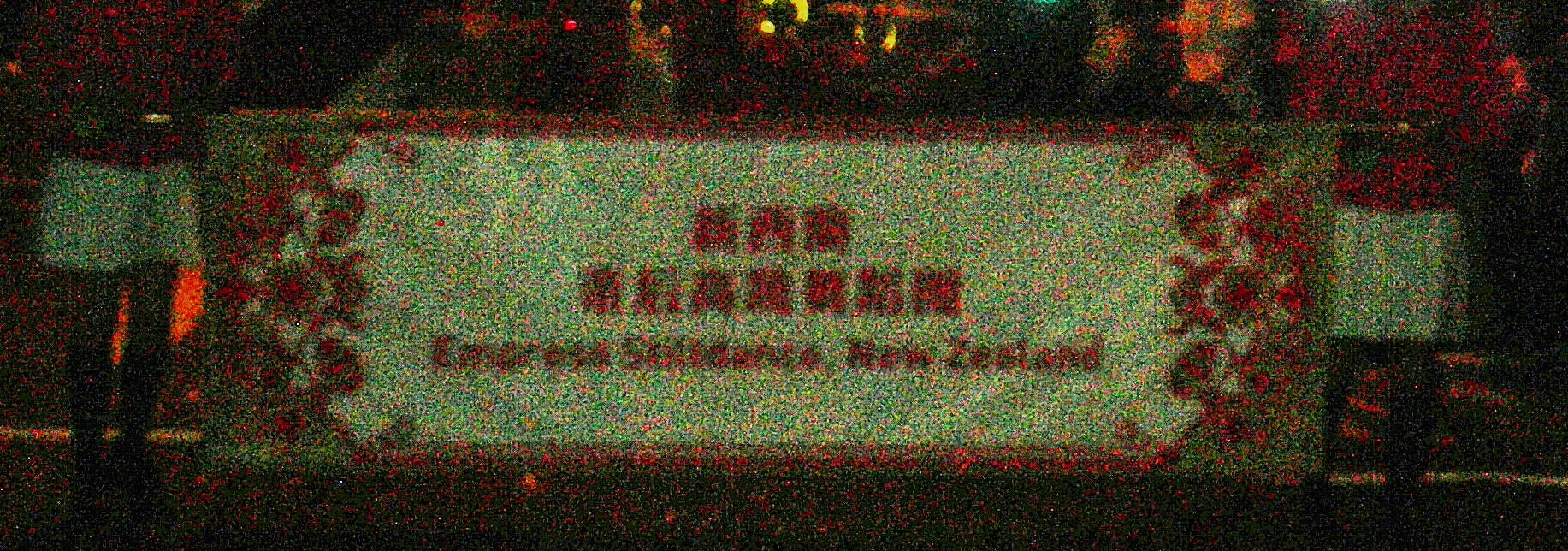The image appears to be a low-quality, blurry photograph taken in poor lighting conditions during a parade-like event, with a dark background and splashes of red, orange, and yellow from other illuminated objects. The focal point of the photo is a horizontal banner held by two people on either side, who are wearing red tops, white skirts or shorts, and long black boots. Their heads are cut off in the image. The banner is suspended from a stiff rod and features a green border with a red filigree design, while its center is white with red lettering that is largely illegible. The text possibly references a location in New Zealand, with fragmented readable parts such as "EMPRO" or "Empress". The background includes a dimly lit street with a yellow line running from left to right.